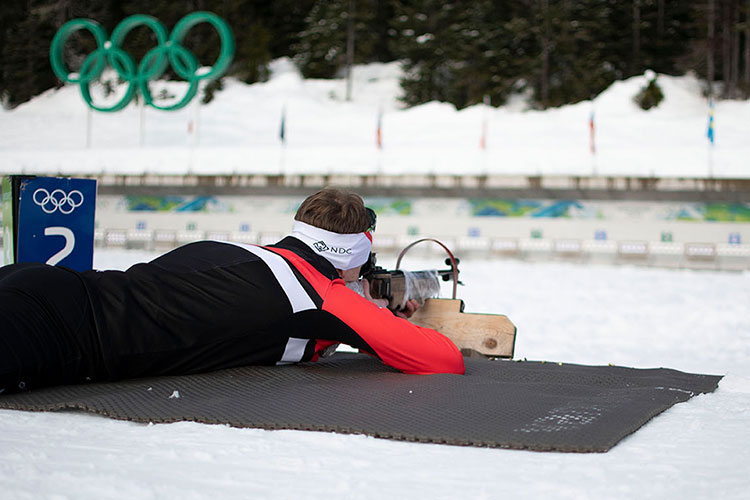This color photograph captures a Winter Olympic shooter in action, lying prone on a dark gray padded mat to shield against the snow-covered ground. The athlete, dressed in a distinctive black, white, and red tracksuit, is aiming their rifle, which is securely perched on a wooden block in front of them. The shooter wears a white headband emblazoned with the letters "NDG." To their left, a blue sign showcases the number '2,' accompanied by the iconic Olympic rings, signifying their competition status. In the blurred background, a snowy landscape with pine trees and a glimpse of stadium seating can be observed, highlighting the cold, wintry setting of this Olympic event.